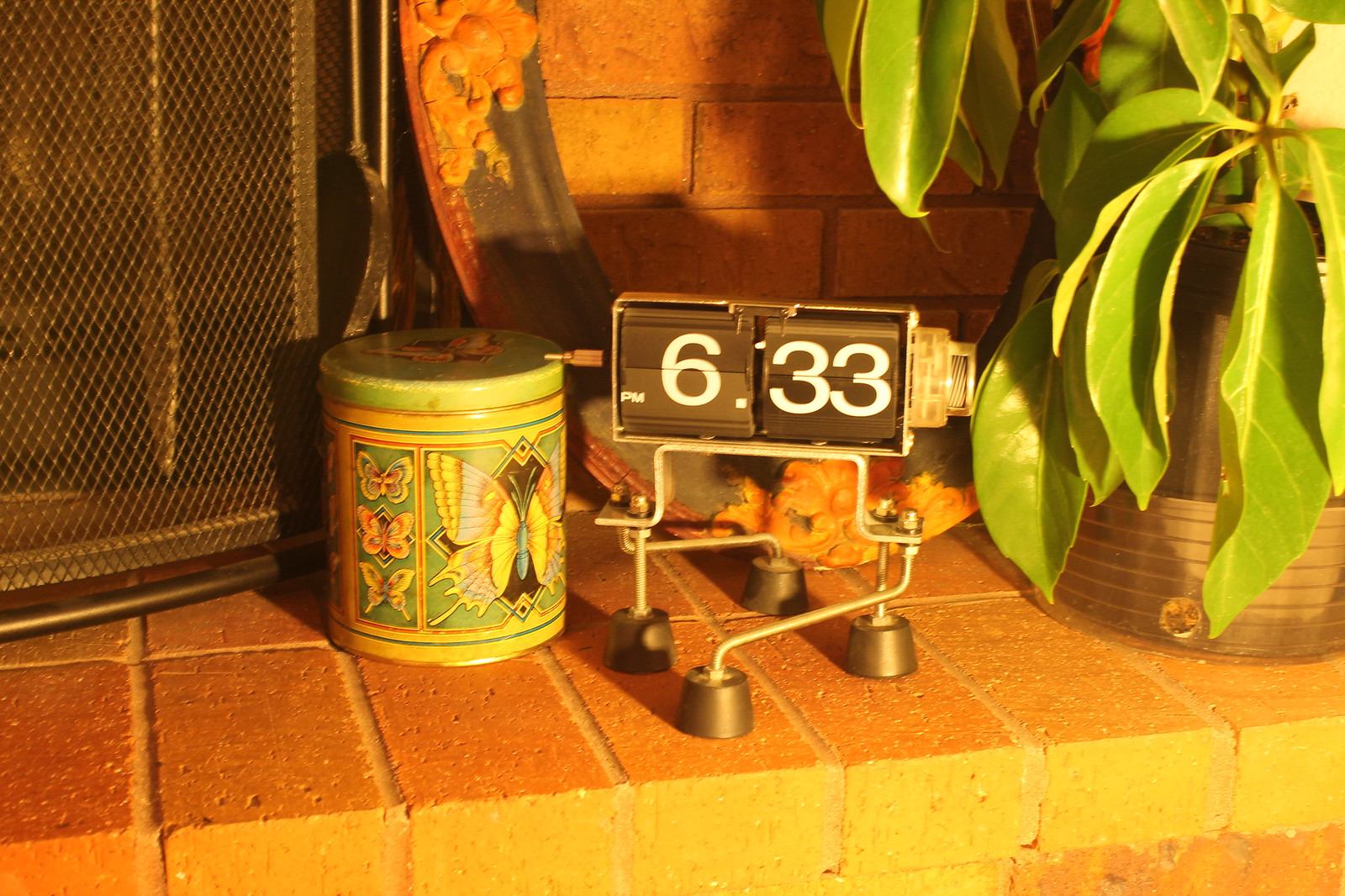This photograph captures the cozy ambiance of a fireplace setting, focusing on the red brick base adorned with various intriguing items. To the left, a black metal grate covers the fireplace, providing a sense of warmth and protection. In front of the grate sits a small, greenish-yellow metal tin adorned with a large butterfly and a vertical row of three smaller butterflies. Beside the tin is a distinctive flip-clock shaped like a pill bottle, displaying the time as 6:33 p.m. This clock rests on unique wire feet, adding a quirky touch to the scene. To the right of the clock, a lush green plant thrives in a black pot, completing the charming and eclectic arrangement on the vibrant brick surface.